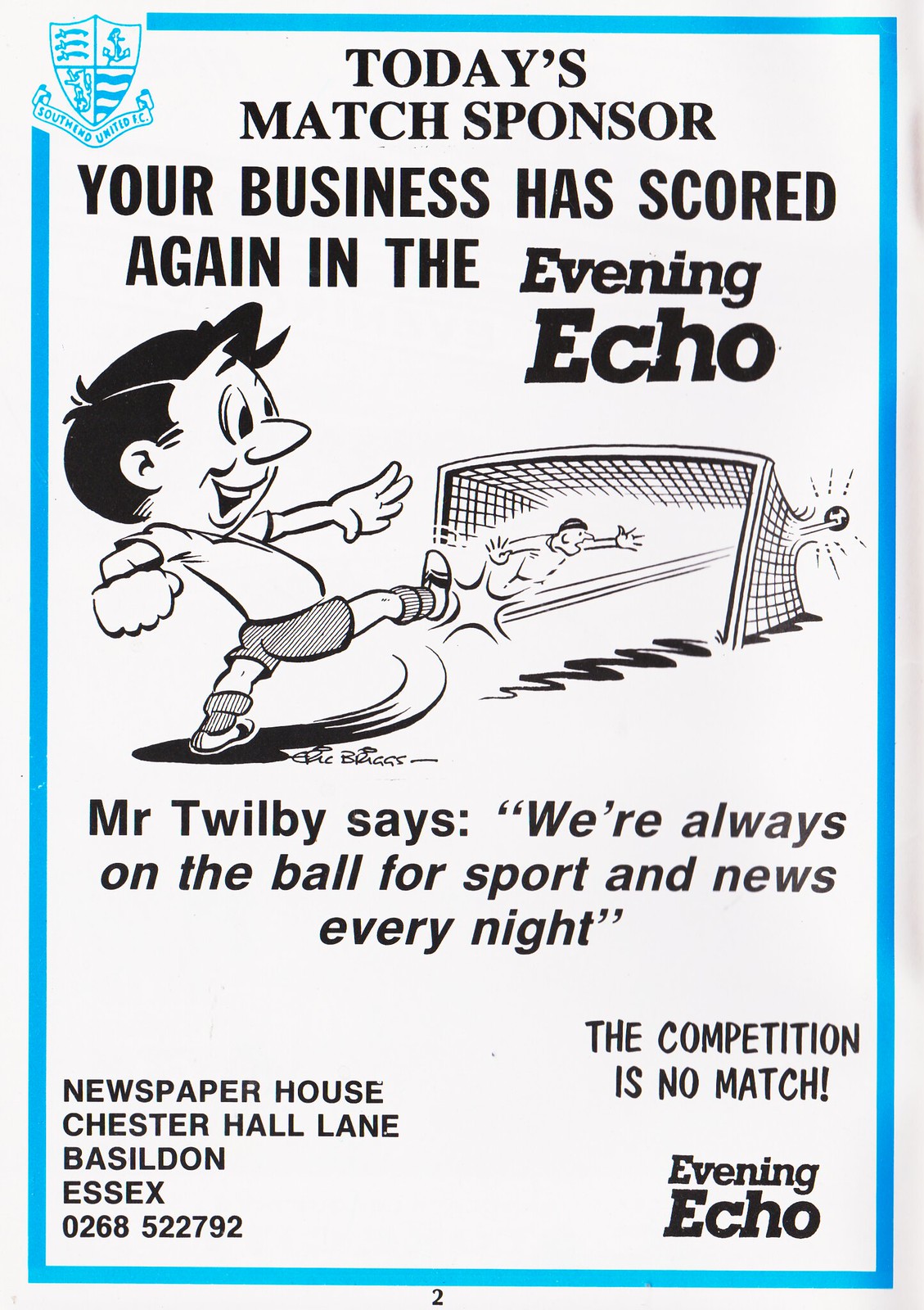The advertisement for the "Evening Echo" is a detailed, full-page illustration with a vivid light blue square border around it, except for the top left corner, which features a badge-like crest with a shield and banner reading "Sutherland United." The page has a clean white background with all the text in black. At the top of the ad, bold text reads, "Today's match sponsor, your business has scored again in the Evening Echo." Beneath this, there is a striking black-and-white cartoon illustration depicting a young boy with black hair energetically kicking a soccer ball through a net, with such force that the ball appears to be blasting through the back of the goal. The goalie is shown with outstretched hands and an open mouth, emphasizing the action. A streaking line traces the path of the ball from the boy's kick to its impact. Below the illustration, a caption reads, "Mr. Twilby says, we're always on the ball for sport and news every night." In the bottom left corner, the contact information lists "Newspaper House, Chester Hall Lane, Basildon, Essex, 0268-522-792." In the bottom right corner, bold text asserts, "The competition is no match," next to the "Evening Echo" logo. The layout is rectangular, taller than it is wide, balancing visual elements and informative text effectively.